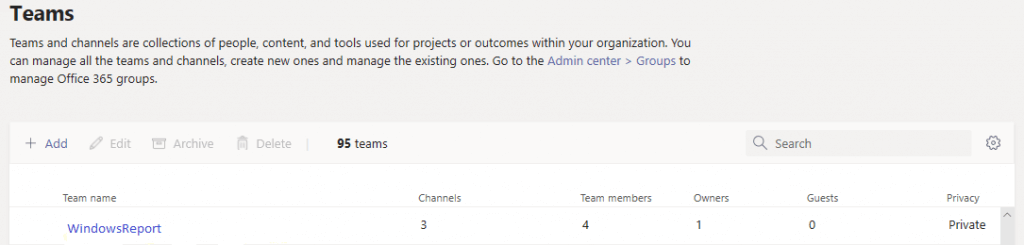Screenshot of the Microsoft Teams Admin Center. Displayed is the management interface for Teams and Channels, showcasing a structured table for organizing groups within an organization. Each "Team" represents a collection of people, content, and tools focused on projects or outcomes relevant to the organization. The table reveals information about a team named "Windows Report" which includes columns for "Team Name," "Channels" (3), "Team Members" (4), "Owners" (1), "Guests" (0), and "Privacy" (Private). At the top of the interface, it indicates there are 95 total teams, although only the "Windows Report" team is visible in this screenshot. This interface allows users to manage existing teams, create new teams, and oversee Office 365 Groups by navigating to the Admin Center and then to "Groups." The display features a light theme with black font, offering clear visibility and organization of information. This is an example of collaboration software that supports team-based communication and management within a company.